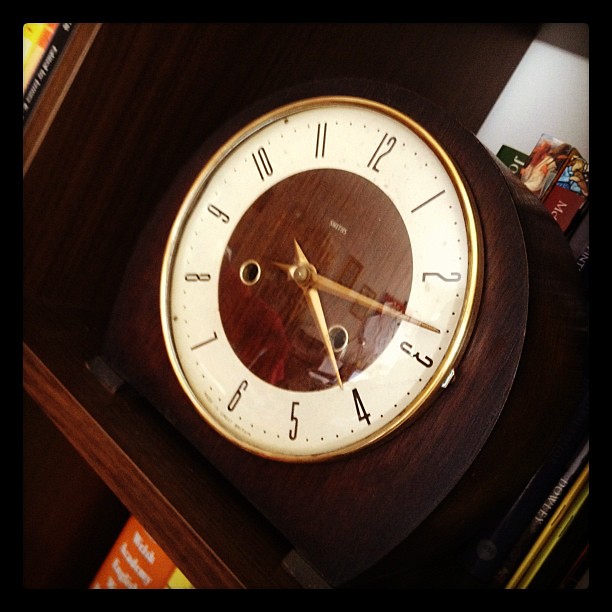The image depicts a vintage or antique clock, presented at a slight tilt, revealing the 11 o'clock mark at the top of the screen for an unusual perspective. The clock is circular, set within an oval-shaped, dark brown wooden frame, and features a gold metal frame around its perimeter. The face of the clock is designed with an outer white border displaying brown numbers from 1 to 12, while the inner circle is dark brown wooden. The gold-brass clock hands indicate the time as approximately 4:12 or 4:13. In the background, the clock is perched atop a bookshelf, with two levels separated by a diagonal wooden plank that extends from the middle left to almost the center of the image. Behind the clock, a dark wooden cabinet or shelving can be seen, featuring various books, including a green one with a white 'J', a red one with a white 'M', and another red book with 'WIF' in white letters partially visible.